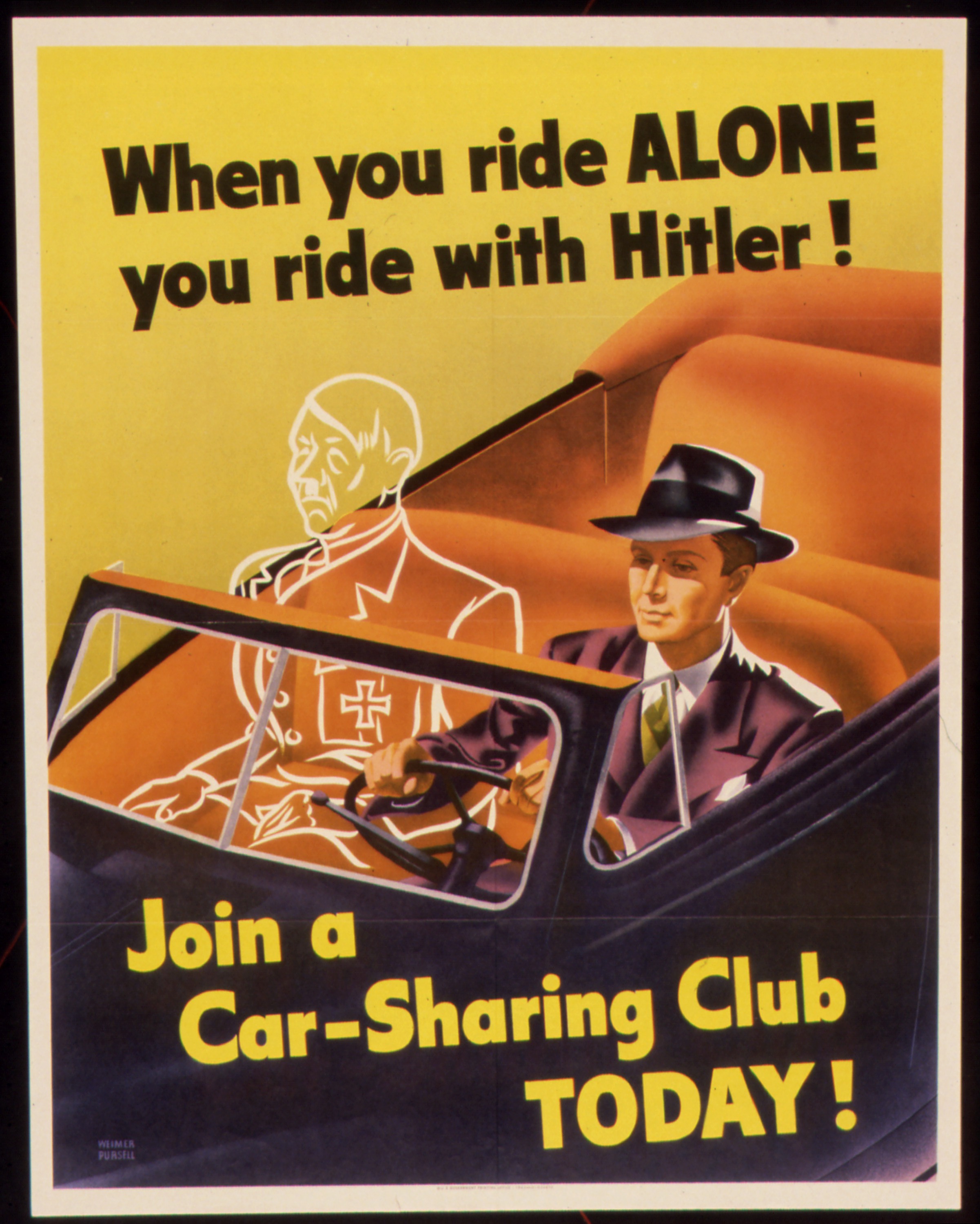The image is a vintage propaganda poster with dimensions akin to a standard sheet of paper, approximately five to six inches high and four inches wide, featuring a thin black frame. Dominating the poster is a backdrop with a vibrant yellow background. Central to the image is an old-fashioned black convertible automobile, angled from the lower left towards the upper right, showing both a front and back bench seat upholstered in orange.

In the driver's seat sits a man dressed in mid-20th century attire: a purple suit, a yellow tie, a white button-up collared shirt, and a gray fedora. To his left, haunting the passenger seat, is a white ghostly outline of Adolf Hitler, depicted with a military uniform bearing a cross symbol on the chest, and hands resting in his lap.

The poster conveys a stark message with bold black text at the top stating, "When you ride alone, you ride with Hitler!" Beneath, against the black of the car, yellow text urges viewers to "Join a car sharing club today!" This image uses striking visual contrast and direct language to promote carpooling during wartime.